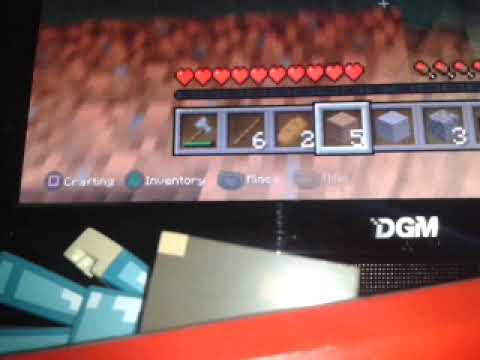The image features a close-up view of a flat-screen TV, displaying what appears to be a Minecraft-style video game. Dominating the screen are several red hearts arranged horizontally, indicating player health, and various inventory slots. Among the inventory items are a block, a weapon, and numerical squares displaying the numbers "6" and "2." Additionally, a mine symbol is visible within one of the squares. The TV brand "DGM" is clearly marked at the screen’s center-right. Below the game's main display, several button commands are listed: "Crafting," "Inventory," "Use" (LT), and "Mine" (RT). The image also includes a partial view of the surrounding interior environment, revealing a wooden piece jutting out from the bottom right corner and some blurry objects in teal and orange, likely thumb drives or similar items.